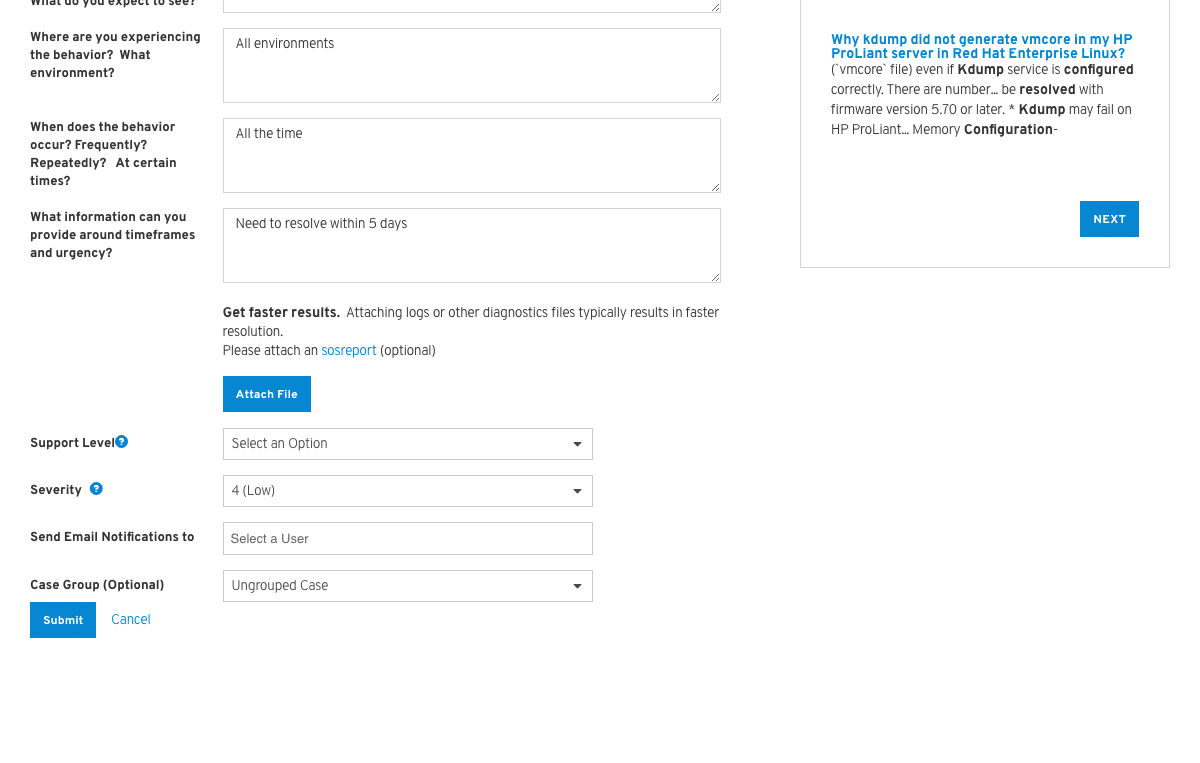This is a detailed screenshot of an unknown support form interface, possibly from a technical support or ticketing system, designed to capture comprehensive issue reports. The form prompts users with multiple questions to detail the encountered issue:

1. **Prompts at the top**:
   - **What do you expect to see?**
   - **Where are you experiencing the behavior?** Options include: All environments.
   - **When does the behavior occur?** Options include: Frequently, Repeatedly, At certain times, All the time.

2. **Additional details requested**:
   - Timeframes and urgency: Need to resolve within five days. 
   - Suggestion for faster results: Attaching logs or diagnostics files typically results in faster resolution.
   - Optional: Attach an SOS report.

3. **Form fields**:
   - Attach file
   - Support level: select an option
   - Severity: four, low
   - Send email notifications to a selected user
   - Case group: optional, defaulting to ungrouped case

4. **Action buttons**: 'Submit' and 'Cancel'.

To the top right corner of the screenshot, a question highlights the specific technical issue: "Why KDUMP did not generate VM Core in my HP ProLiant server in Red Hat Enterprise Linux?" It notes that even with the KDUMP service configured correctly, the VM Core file may not generate, possibly resolvable with firmware version 5.7 or later. KDUMP may fail on HP ProLiant memory configurations.

There is a blue "Next" button at the bottom of the form.

The image is entirely textual with no photographic elements. It includes no visual images of people, animals, birds, plants, flowers, trees, or automobiles.